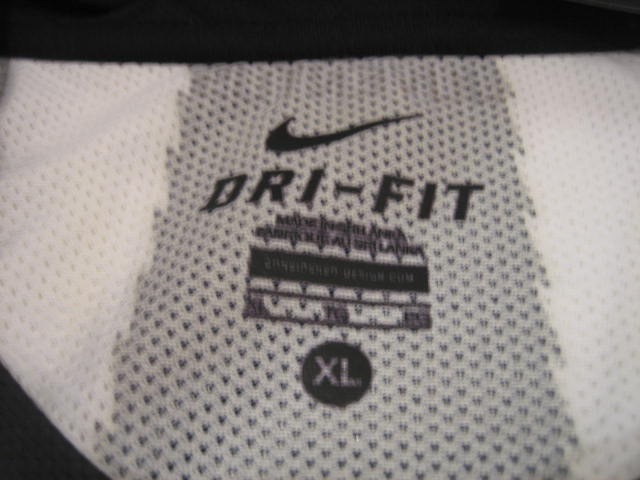The image is a close-up of a piece of sportswear fabric, likely a Nike Dri-FIT item. The fabric features a combination of white and gray colors, arranged with a white strip on the left, a gray middle section, and another white section on the right. The Nike logo, a black curved checkmark, is prominently displayed at the top of the gray section. Below the logo, the words "DRI-FIT" are screen printed in large letters. Further down, there is additional smaller text indicating that the item is made in Sri Lanka. Centrally positioned at the top of the fabric, there is also a black circle with "XL," denoting that it is an extra-large size. The fabric appears to have a knit pattern with small breathable holes throughout, enhancing its functionality for sportswear.